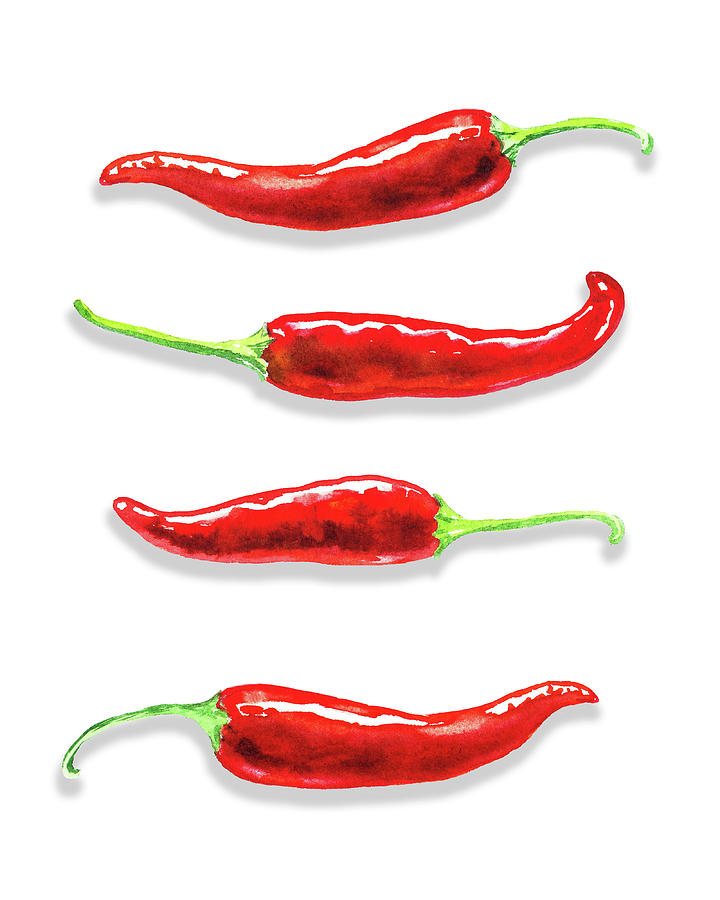This image depicts a detailed illustration of four red chili peppers with green stems, positioned vertically from top to bottom against a white background without a border. Each chili pepper alternates in direction, with the top pepper's stem pointing to the right, the next to the left, and so forth. The peppers lie in a row, each casting a subtle drop shadow on the white surface beneath them. The stems of the peppers are long, thin, and slightly curled at the tips, consistent with the light source coming from the top of the image, casting a white highlight on the upper side and a darker shadow below. Notably, the peppers are not uniform in shape; the third pepper is distinctly smaller and stubbier than the others.